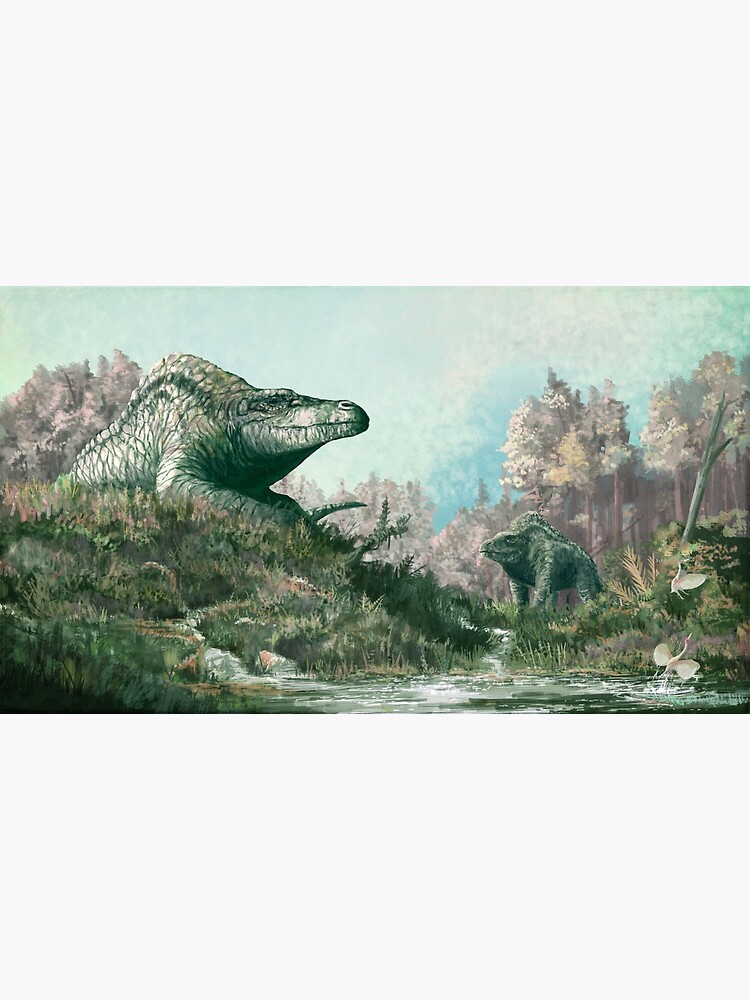The image depicts a detailed rectangular painting from the dinosaur era, focusing on a lush prehistoric landscape. Two green-scaled dinosaurs dominate the scene; the larger one on the left is walking towards the right, while the smaller one on the right moves to the left, creating a dynamic balance within the composition. The ground is a rich green with abundant vegetation, and a water body, possibly a small lake or pond, lies at the bottom. The background features numerous light pink trees, adding a striking contrast against the bluish-green sky. The painting itself is enclosed within a frame where the top and bottom sections include light gray horizontal strips, making up about 40-45% of the overall image space. This illustration vividly captures a moment in deep prehistoric past, blending naturalistic detail with a slightly green-tinted atmosphere to bring the ancient scene to life.